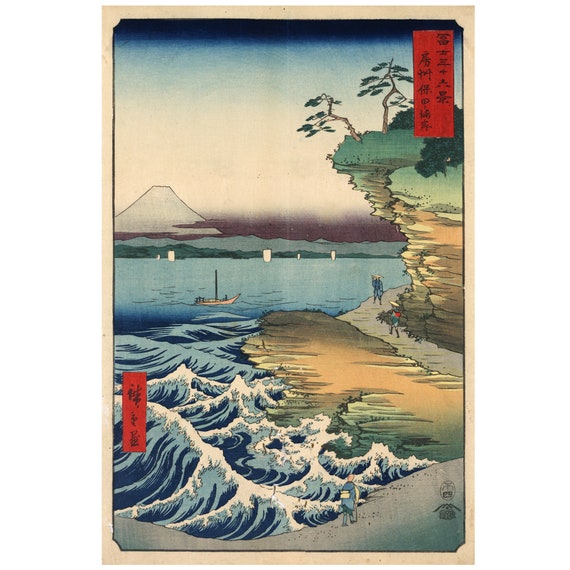The image is a color print or poster depicting a Japanese shoreline scene. On the left-hand side, Mount Fuji, a prominent white mountain, stands majestically against a gradient sky transitioning from white to dark blue. Below Mount Fuji, a calm blue body of water stretches across the center of the image, dotted with a simple sailboat and more sailboats further in the distance. The body of water varies in texture, with white-capped waves appearing in the lower left corner, transitioning to calm water under a cliff on the right side.

This cliff, which is brown with jagged edges, rises to reveal a green, grassy top adorned with a few trees. Below the cliff, a path runs parallel to the water, where people can be seen walking near the coastline. In the lower right corner, more jagged waves suggest rougher water. Additionally, the image features rectangular areas with black text, one in the upper right corner and another in the bottom left. There are red boxes with Japanese characters adding to the traditional aesthetic of the print.